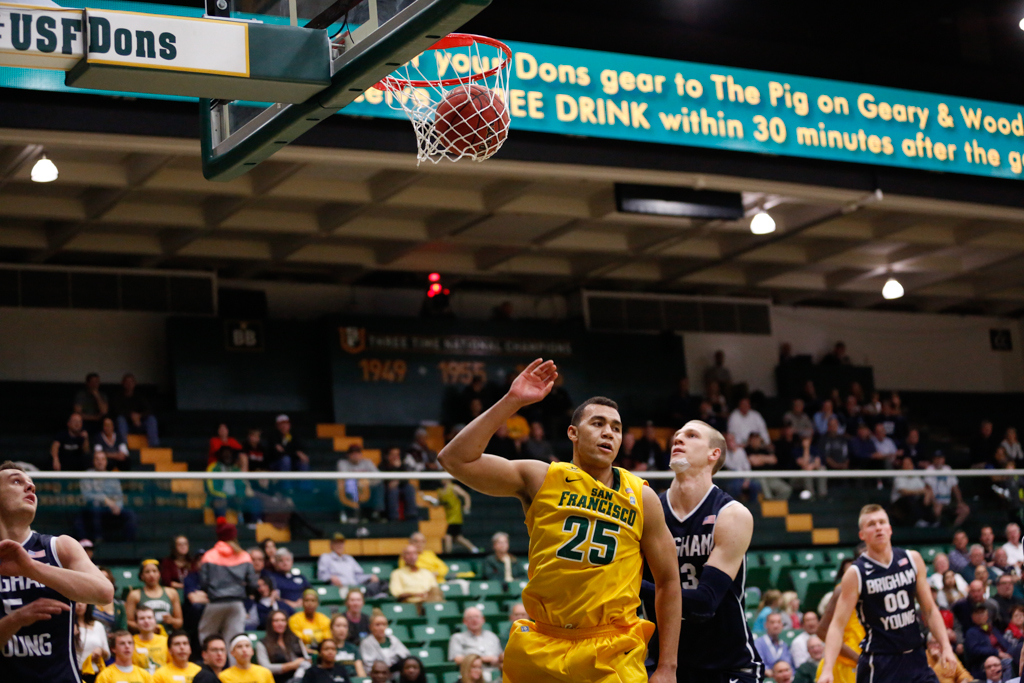This color photograph captures an intense moment during a men's basketball game between the University of San Francisco (USF) and Brigham Young University (BYU). The focal point of the image is number 25 from San Francisco, dressed in a gold uniform with green trim and the Nike logo on his right chest, having just shot a basket. The ball is mid-fall inside the net, which is oriented to the right side of the frame. Surrounding him are four other players: three from BYU in navy blue uniforms with white trim and another USF player also in gold. The arena's background reveals a blend of green seats and bleacher sections with a mix of empty seats and spectators, some of whom are wearing gold. A digital advertisement spans the top of the image, promoting "Don's gear to the pig on Geary and Wood" with a special offer for a free drink within 30 minutes after the game. The structure supporting the hoop prominently displays "USF Dons."